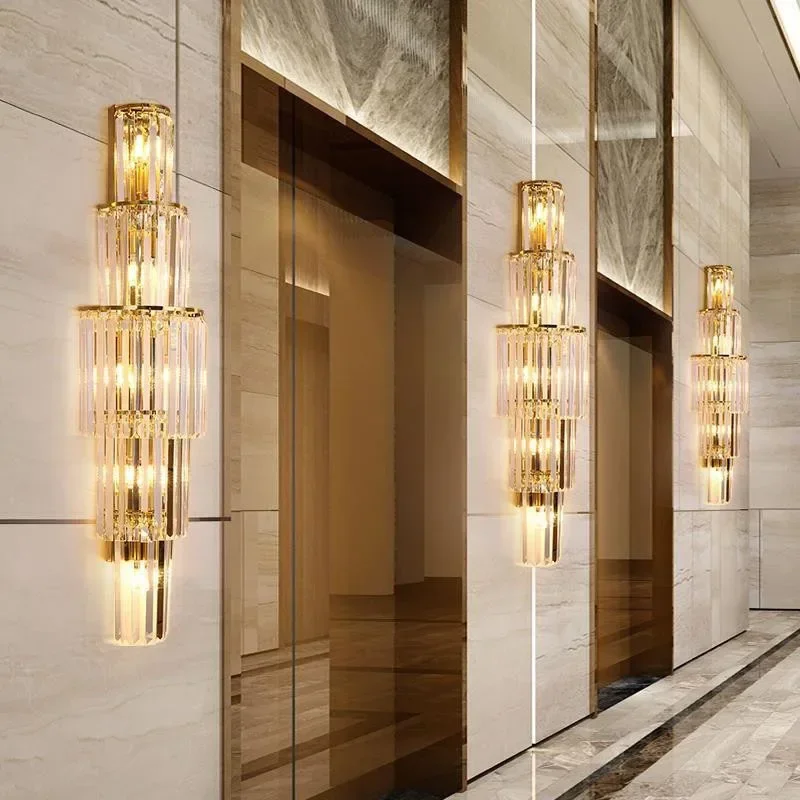The image depicts a luxurious and immaculately clean building interior, featuring two prominently positioned brown elevator doors flanked by golden chandelier lights. The setting exudes opulence with its beige and grey tile walls accented with gold and touches of brown. The elevator doors, with their gleaming bronze finish, are complemented by intricate ornamental lighting on either side and between them, featuring small bulbs and crystals that create a dazzling effect as they reflect light in multiple directions. The ceiling is pristine, enhancing the overall brightness of the area, which benefits from ample lighting. Above the elevators, marble inlays display their distinct grain, adding an extra layer of sophistication. The floor is covered in shiny, large grey tiles with dark grey accents, contributing to the sleek and modern aesthetic of the space.